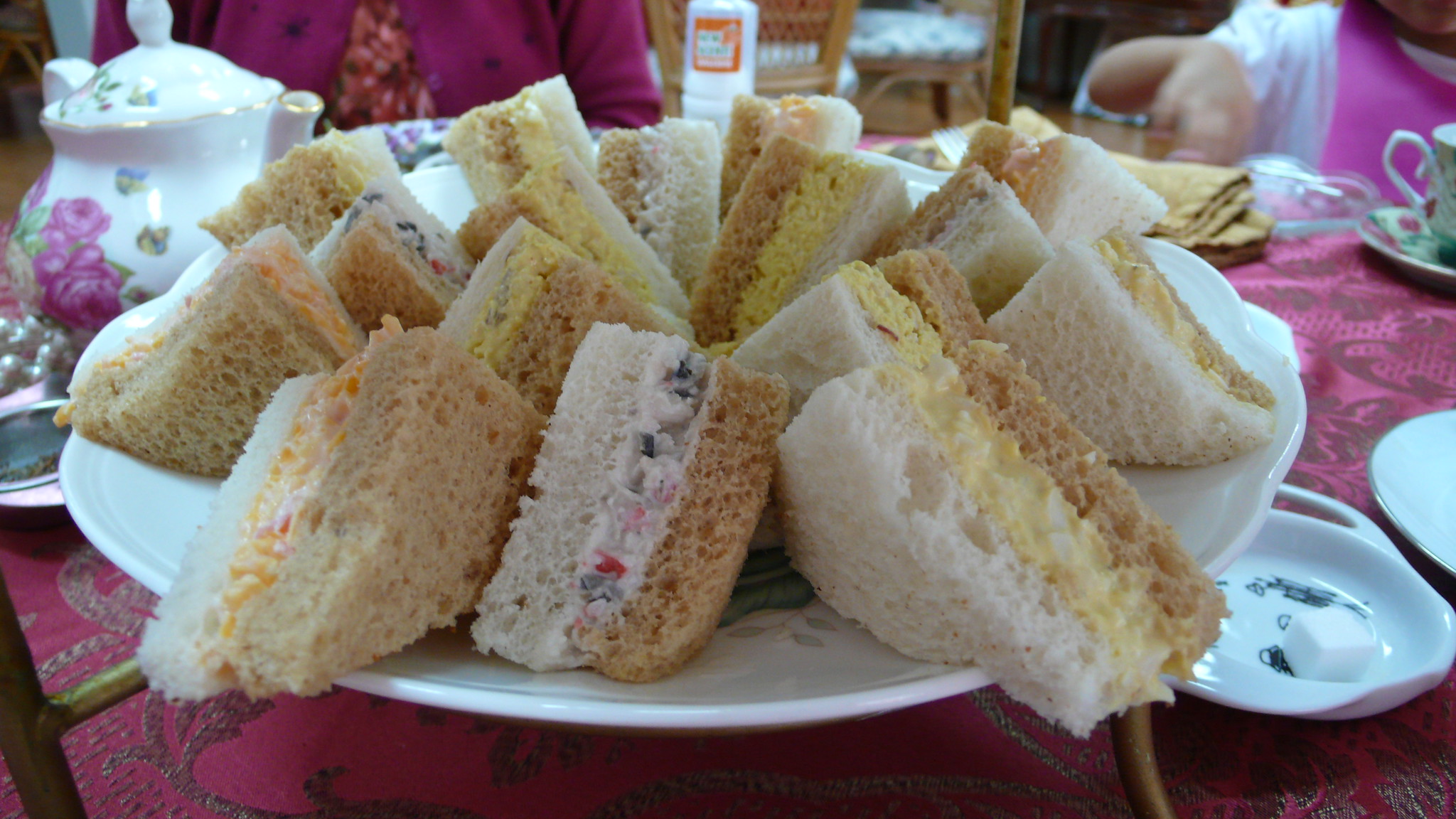This close-up, horizontally oriented photograph captures a charming scene of finger food sandwiches meticulously arranged on a white scalloped ceramic plate. Each sandwich is composed of either two layers of white bread, or a combination of white and brown bread, and cut into perfect little triangles. The fillings include egg salad, pimento cheese, and possibly chicken salad, featuring colorful ingredients like peppers and cranberries. The crusts have been delicately removed, enhancing the neat, artistic presentation.

The plate sits on a decorative table adorned with a maroon tablecloth featuring green and olive floral embroidery and is complemented by an array of fine china. This setup includes a teapot with floral designs, teacups, and saucers. In the background, there's a suggestion of an outdoor, tranquil setting, perhaps on a slightly overcast day, creating a soft blueish hue across the scene.

The photograph also captures the hands and partial images of two individuals - one wearing a maroon-colored shirt and the other with olive skin in a white shirt with a pink bib - suggesting an inviting tea party atmosphere. The ambiance is further enriched by gold napkins and additional ceramic platters, making this a cozy and refined yet accessible setting perfect for both children and adults.